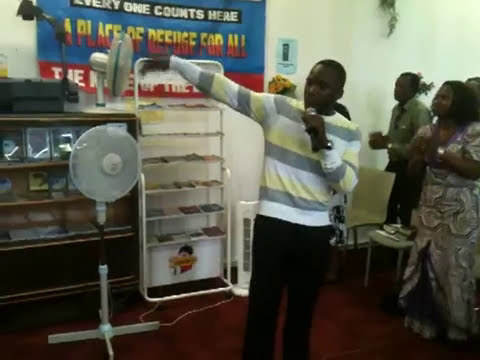In this detailed indoor photograph set within a school or institution, a bald black man in his 20s or 30s, dressed in a long-sleeved sweater with white, gray, and yellow horizontal stripes, stands holding a microphone with a silver head in his left hand, while his right hand gestures upwards towards the top left corner. The man, who is wearing black pants and a watch on his left wrist, appears to be addressing an audience or conducting a lecture. Behind him on an off-white wall, a colorful banner reads, "Everyone Counts Here, A Place of Refuge for All." To his left, the room features a bookcase and a shelf holding various items, possibly CDs, while a floor-mounted fan stands nearby. On his right, two black women are present: one in a long, white and purple floor-length dress with shoulder-length hair, and the other in a denim shirt. The setting includes a dark red carpeted floor and additional shelves adorned with photo frames, books, and possibly a briefcase.